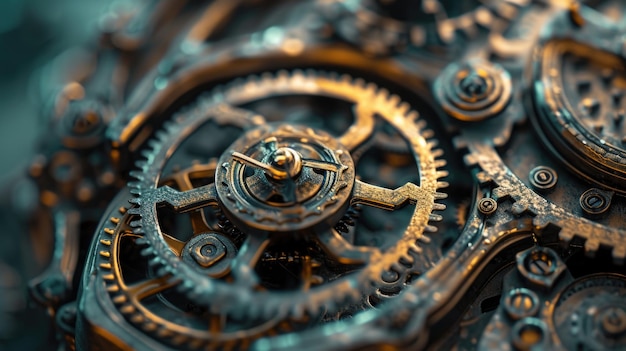The image is a highly detailed, close-up view of a series of interconnected gears, reminiscent of the intricate inner workings of an old-fashioned watch or clock. The predominant focal point is a large, centrally positioned gear with a tarnished gold exterior and small nubs around its circumference. This central gear features several arms extending from a rounded center to the outer edge, where the points or teeth are visible. Surrounding this main wheel are numerous other gears, which appear stacked and interconnected, gradually fading into a blur towards the background. The overall color palette of the gears includes metallic tones such as brass, copper, and tarnished silver, mixed with patches of dark gray and hints of a teal patina, adding an antique, steampunk aesthetic. The background, especially noticeable in the upper left corner, blends dark shades of black, gray, and blue, further amplifying the focus on the gears. The image, which appears to have an artificially generated or digitally designed quality, emphasizes the mechanical complexity and visual appeal of these interlocking components.